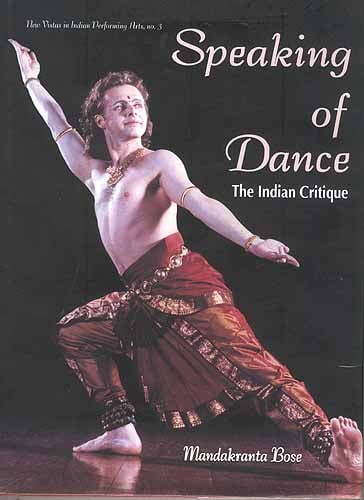The image features an advertisement, possibly for a book or magazine, with a dark brown background. Prominently displayed is a photograph of a young man engaged in a traditional Indian dance pose. He is bare-chested, adorned with a gold necklace, and has various bracelets on his wrists and biceps. His attire consists of maroon-colored pants with gold trim, extending down to his bare feet. His right leg is bent to the side in a plié position, and his left foot is flat on the ground. He has long, wavy brown hair and a jewel or traditional mark on his forehead.

His arms are elegantly outstretched, one pointing upward and the other outward with a finger extended. His gaze is directed upwards as if looking towards the sky. The text "Speaking of Dance, The Indian Critique" appears in white, cursive letters along the top right of the image. The name "Mandakranta Bose" is written at the bottom, also in white cursive, placed near his left leg. In the upper left corner, additional information is provided in white text, giving more context to the image, enhancing its purpose as a visually striking promotional piece for an event or publication focused on Indian dance.